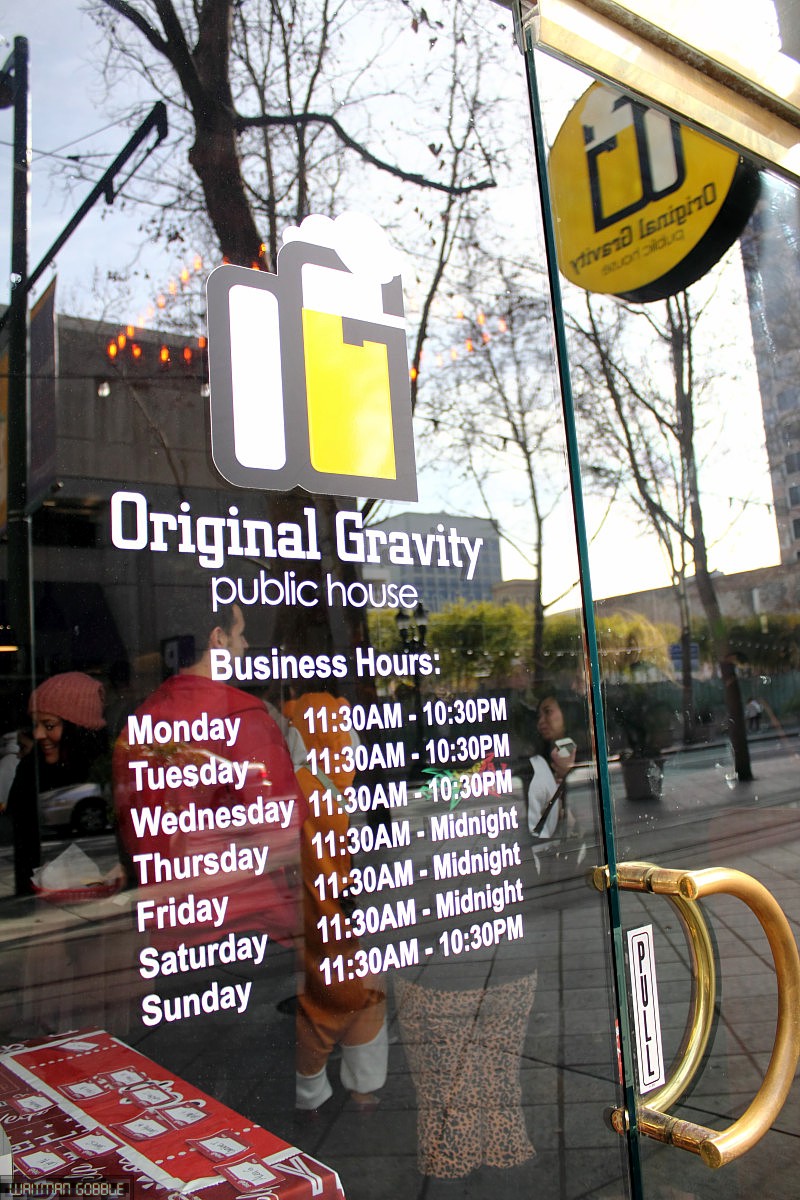This outdoor daylight color photograph captures the front entrance of The Original Gravity Public House, featuring a prominent glass door with a curved gold handle. Adhered directly to the door is a detailed emblem and text, starting with an OG logo. The 'O' is represented as a white vertical column, while the 'G' resembles an overflowing beer mug with what appears to be yellow liquid and white frosting at the top. Beneath the logo, white text reads "Original Gravity Public House." Below that, the business hours are listed: Monday through Wednesday, 11:30 a.m. to 10:30 p.m.; Thursday through Saturday, 11:30 a.m. to midnight; and Sunday, 11:30 a.m. to 10:30 p.m. 

Further details include the reflection of the street, city buildings, and trees seen on the glass surface. There's also a white sticker with the word "PULL" in black letters affixed to the gold handle. Inside the establishment, a red tablecloth with white decals is visible on a table in the bottom left corner. Two people are discernible—one wearing a red jacket and another person in an orange outfit, both standing near a counter.